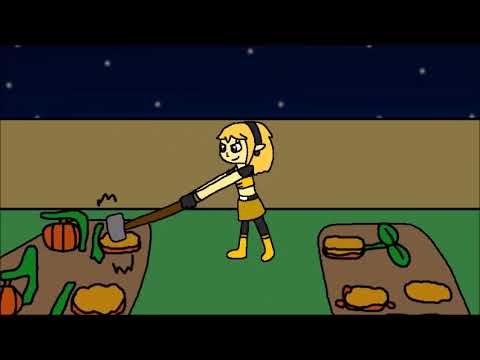This is a pixelated, hand-drawn cartoon image resembling a screenshot from an old video game. It features a teenage girl positioned centrally, with fair skin and blonde hair tied back with a black hairband. She wears a yellow dress that reaches her knees, paired with a black t-shirt, black leggings, and yellow boots. The girl's face is turned to the left, displaying a mischievous expression as she wields a sledgehammer. She is in the act of smashing objects, likely pumpkins, placed on the green ground which resembles a lawn. To her right, already shattered remains are visible, while to her left, some intact pumpkins await their fate under her hammer. The scene is set against a dark navy blue sky dotted with stars, divided by a horizontal brown strip that could represent a wall or tablecloth. The top and bottom of the image are framed by horizontal black strips, suggesting a digital screenshot or an animation frame. The setting exudes an air of nighttime mischief in a garden-like area.